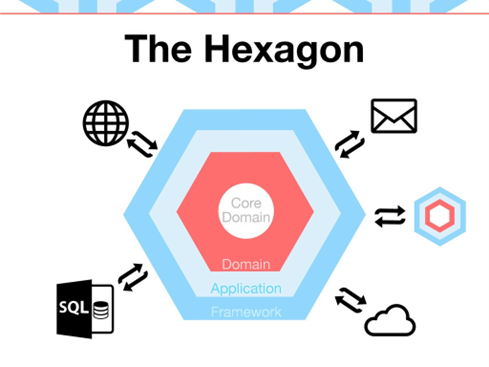The image, titled "The Hexagon," is a detailed, multi-layered hexagon on a white background with black lettering. The central design showcases three nested hexagons: the outermost hexagon has a blue border, the middle one is light blue, and the innermost hexagon is rose-colored, with a small white circle at the core. The core circle contains the words "core domain" in very light gray letters. Above the hexagon in black letters is the title "The Hexagon."

Surrounding the central hexagon are five smaller black-and-white images, each connected with double-headed arrows indicating interaction. These images include: an envelope at the top right, a smaller replica of the central hexagon to its right, a cloud at the bottom right, a globe with crisscrossed lines at the upper left, and an open book labeled "SQL" at the bottom left. Above the title text "The Hexagon," there are additional blue and white elements. The varying colors used within the hexagon itself—blue, light blue, and rose—contrast with the predominantly black-and-white icons and text, providing a clear and structured overview of a computer application's workings, detailing its core domain, domain, application, and framework layers.